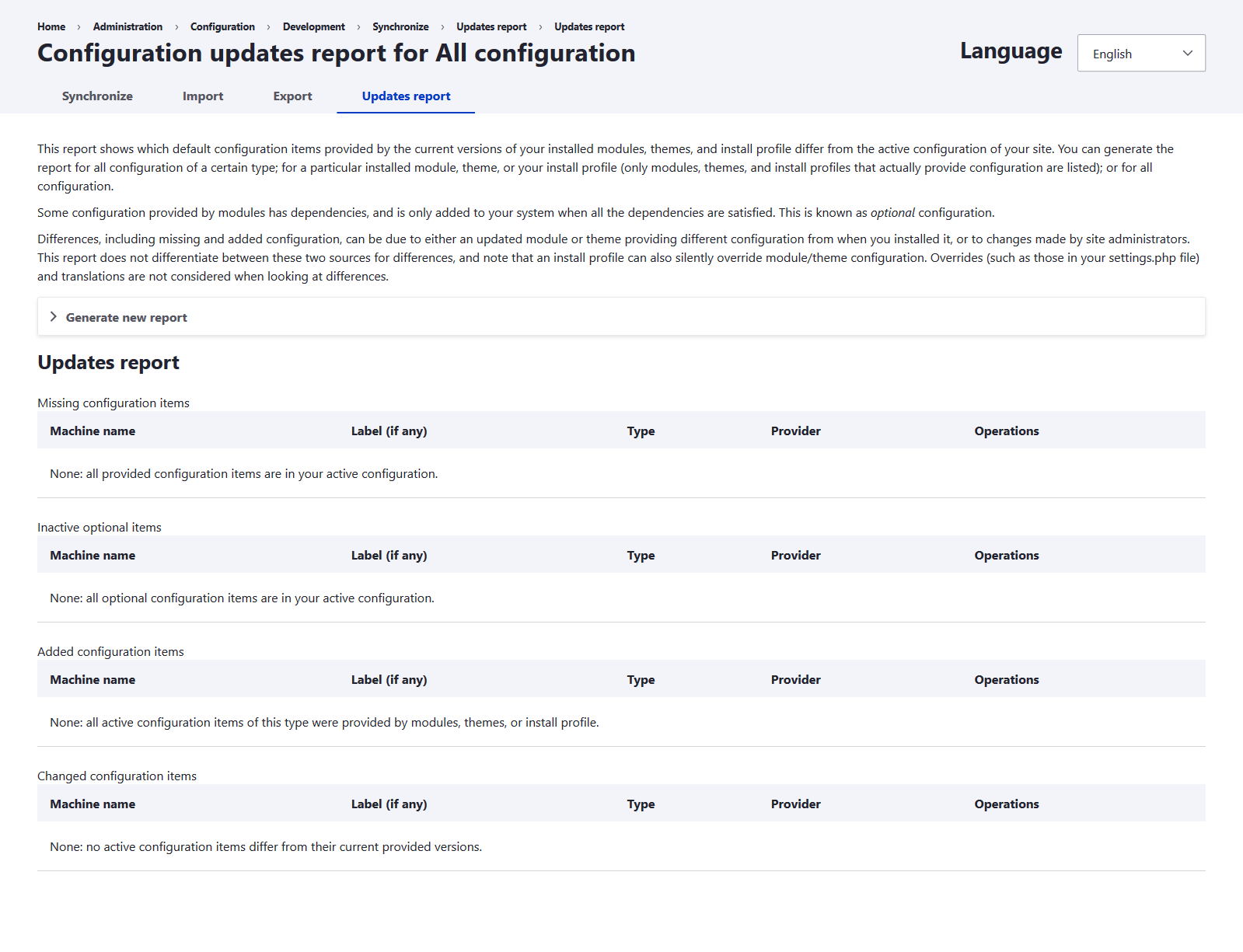This is a screenshot from a website featuring a detailed configuration update report. The top section, approximately an inch and a half in height, is light blue, with the remainder of the background in white. In the top-left corner, there are very small navigation links labeled "Home," followed by arrows pointing to "Administration," "Configuration," "Development," "Synchronize," "Updates Report," and "Updates Report" again.

Beneath these links, in larger bold black text, the heading reads "Configuration Updates Report for All Configuration." To the right, there is an option labeled "Language" with a white tab displaying "English" in black text.

Below the configuration heading still within the blue section, there are links labeled "Synchronize," "Import," and "Export" in black, with "Updates Report" in blue and underscored by a blue line. 

In the white section, the document continues with two paragraphs of textual information, followed by a thin gray rectangle outlined by a gray border. This rectangle includes a right-pointing greater-than symbol and the text "Generate New Report" in black. Below it, there's the title "Update Reports" and a subtext in smaller lettering that reads "Missing Configuration Items."

Further down, spanning the width of the page, a gray rectangle lists column headers: "Machine Name," "Label (if any)," "Type," "Provider," and "Operations." Underneath it says "None. All provided configuration items are in active configuration."

Next, there are sections labeled "Inactive Operation Items," "Added Configuration Items," and "Changed Configuration Items." Each title is followed by a blue bar with identical column headers as above. The content beneath each blue bar mirrors that of the first section, indicating that there are no additional configuration items or changes.